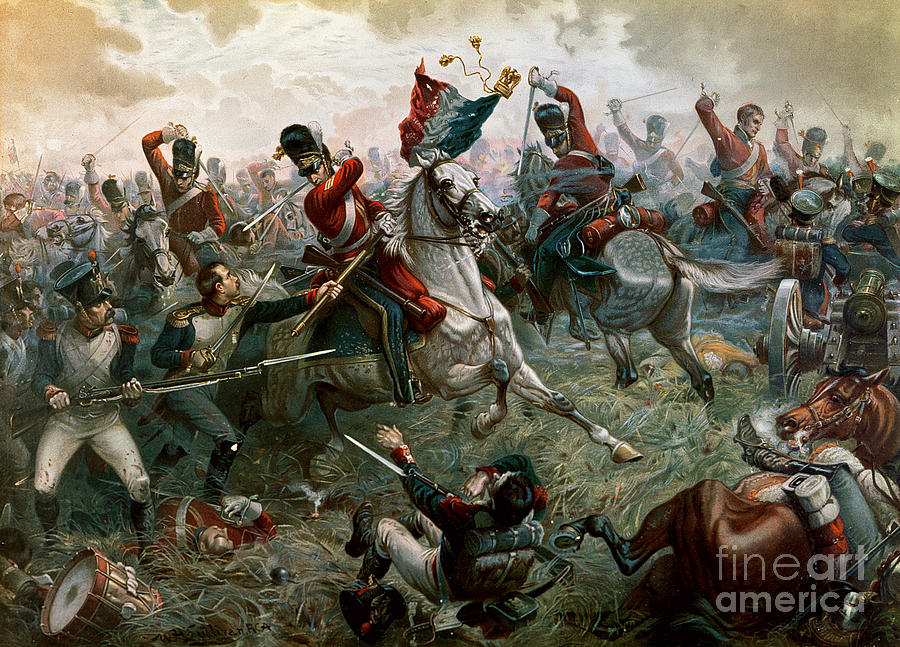This vibrant painting or print depicts a chaotic war scene from the 1800s, likely during the American Revolutionary War, with vivid historical detail. In the battleground, soldiers clad in distinctive red and white uniforms and tall, black hats engage fiercely. Some are on horseback, while others, wielding swords and bayonets, fight on foot. The battle also includes turquoise green uniformed soldiers and one brown horse prominently featured on the right side of the image. Scattered across the ground are musical instruments, including a drum, and a fallen cannon, adding to the scene's authenticity. The backdrop features a light brown sky blending with white clouds, capturing the tumultuous atmosphere of the battlefield. Notably, at the bottom right-hand corner, there is a fine purple text that reads "Fine Art America," subtly marking its authenticity.